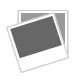The image is a tall, vintage-style poster with a worn and aged appearance, featuring a textured blue-green background. At the top, in bold white capital letters, the text reads: "She was a witch all the time, not just in the reason of pumpkins and crisp leaves." At the bottom, it concludes with: "But always and forever to the depths of her soul."

Central to the image is the sketch of a woman, possibly a young girl, depicted in sepia tones. She is standing with her back to the viewer, reaching upwards with her hand towards an array of celestial elements above her. Her long, sleeveless dress flares out at the bottom, and her hair is styled in a bun. Above her head, a series of moon phases form a triangular pattern, with each moon adorned with various flowers. The full moon prominently features a sunflower, while the other phases display flowers in shades of red, yellow, and pink. The thoughtful composition portrays a blend of mysticism and femininity, encapsulating the thematic essence of the text.